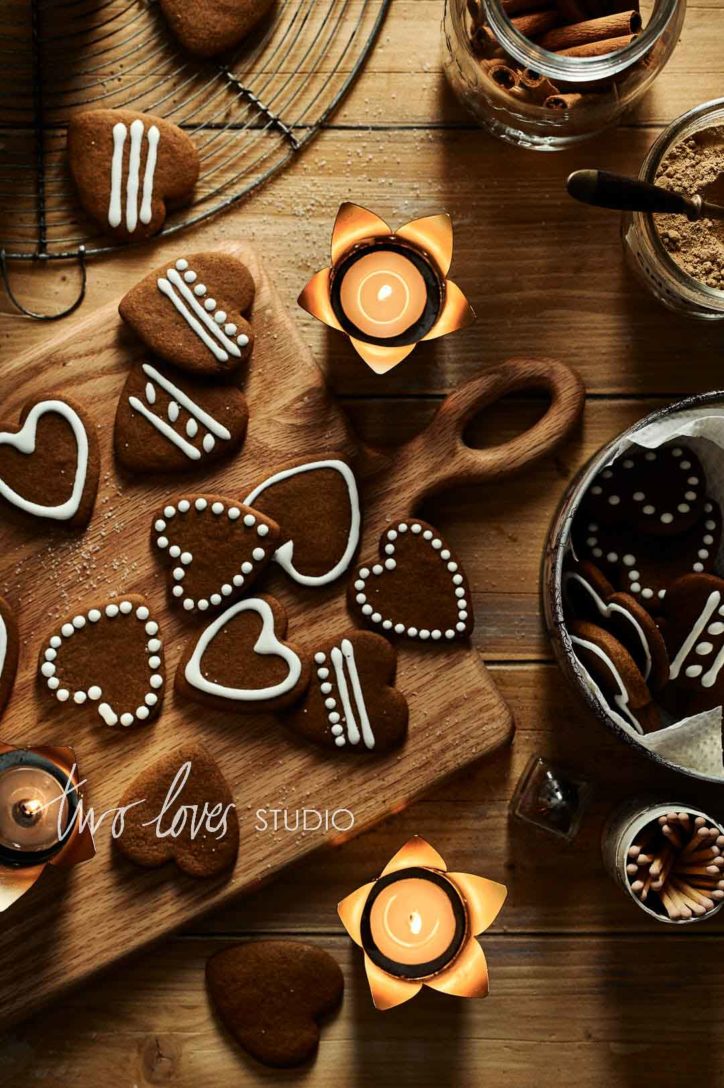The image captures a rustic, naturally aged wooden surface, possibly a table or floor, with horizontal paneling. Spread across this wooden background are various baking-related items, centering on a wooden cutting board that occupies a significant portion of the frame. On the upper left corner sits a circular metal cooling rack, while on the right edge are an assortment of jar tops and containers, including a jar of cinnamon and another unidentified ingredient jar. Scattered around are three tea light candles in flower-shaped holders, casting a warm glow.

At the heart of the setup are dark brown, heart-shaped cookies, meticulously decorated with white royal icing in patterns of lines, outlines, and dots. These cookies are artistically arranged on the cutting board, with some also placed on the cooling rack and inside a decorative tin, likely intended for gifting. The overall color scheme is a harmonious blend of wood brown tones, from the surface to the cutting board and cookies, evoking a cozy, homemade feel.

This is an advertisement for the "Two Loves Studio Cookie Extravaganza," as noted in the printed text on the ad, highlighting the detailed and heart-themed cookie creations.